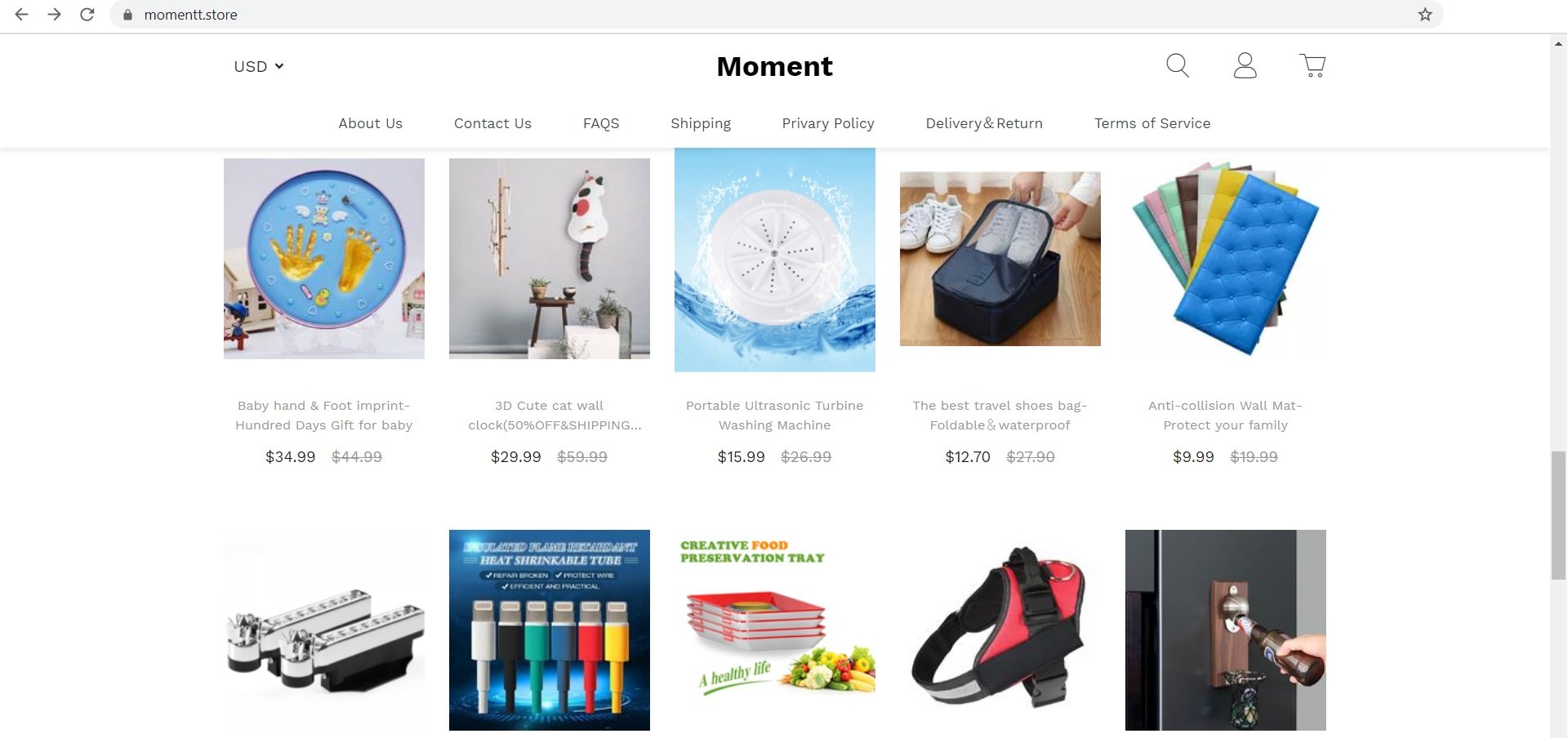This is a detailed screenshot of an e-commerce website interface. The predominantly white webpage features the brand name "Black Moment" prominently centered at the top. On the upper left corner, there's a currency selection labeled "USD" accompanied by a drop-down arrow. On the upper right, there are three icons: a magnifying glass for search, a user profile icon, and a shopping cart icon.

Beneath the brand name, there is a navigation bar with links to various sections including About Us, Contact Us, FAQs, Shipping, Privacy Policy, Delivery, and Terms of Service. 

The main content of the page showcases a grid of products, arranged in two rows with five items per row. One product is a blue circular item resembling a plate, adorned with a gold baby hand and footprint design. Another product is a wall decoration featuring a cat silhouette in gray against a gray background. There is also a portable ultrasonic turbine washing machine clearly visible among the listed items. Additionally, the selection includes a flexible storage bag or box designed to hold shoes.